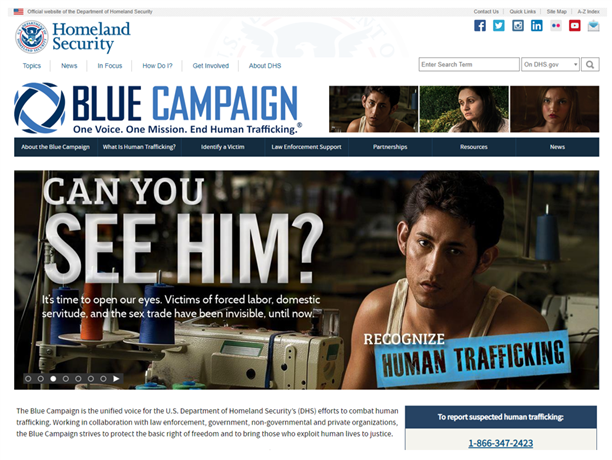The screenshot depicts the official website of the Department of Homeland Security. At the top, there is a small, thin banner featuring the US flag and indicating that this is the official website of the Department of Homeland Security. On the right-hand side, the banner includes navigation options such as "Contact Us," "Quick Links," "Sitemap," and "A-Z Index."

Below the banner, the website displays the Department of Homeland Security emblem with the title "Homeland Security" prominently featured. To the right of the emblem, social media icons for Facebook, Twitter, LinkedIn, and YouTube are displayed.

The site's main navigation menu is positioned to the left and includes sections for "Topics," "News," "Focus," "How Do I?", "Get Involved," "About DHS," and a search bar with a drop-down menu labeled "Search on dhs.gov."

Further down the page, a blue campaign section catches the eye. It includes headings such as "One Voice, One Mission," and "Human Trafficking," accompanied by three individual photos. A dark blue banner beneath this section contains links to "About the Blue Campaign," "What is Human Trafficking," "Identify a Victim," "Law Enforcement Support," "Partnerships," and "Resources."

Prominently featured is a larger banner with a picture of an individual, and the text "Can You See Him?" in white print. The accompanying message reads, "It's time to open our eyes. Victims of forced labor, domestic servitude, and the sex trade have been invisible until now. Recognize human trafficking."